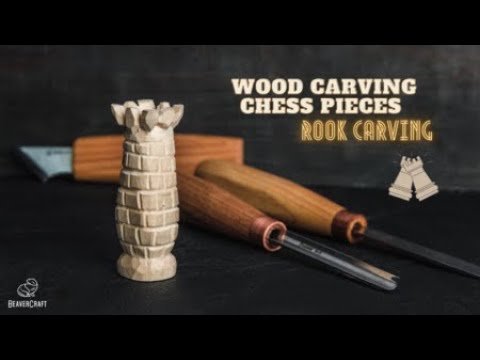The image is a detailed promotional graphic for Beavercraft, a woodcraft tool company. It prominently features a cream-colored rook chess piece crafted from wood, positioned towards the left side. The background includes a variety of wood carving tools: several chisels with brown handles and metal tips, arranged alongside a box cutter also with a wooden handle. The text, displayed in white and brown, reads "Wood Carving Chess Pieces, Rook Carving" and is accompanied by an illustrative logo with two rooks beneath the wording. This composition suggests a technical and sophisticated style appropriate for a sales catalog, highlighting both the intricacy of the woodcarving projects and the quality of the tools provided by Beavercraft.